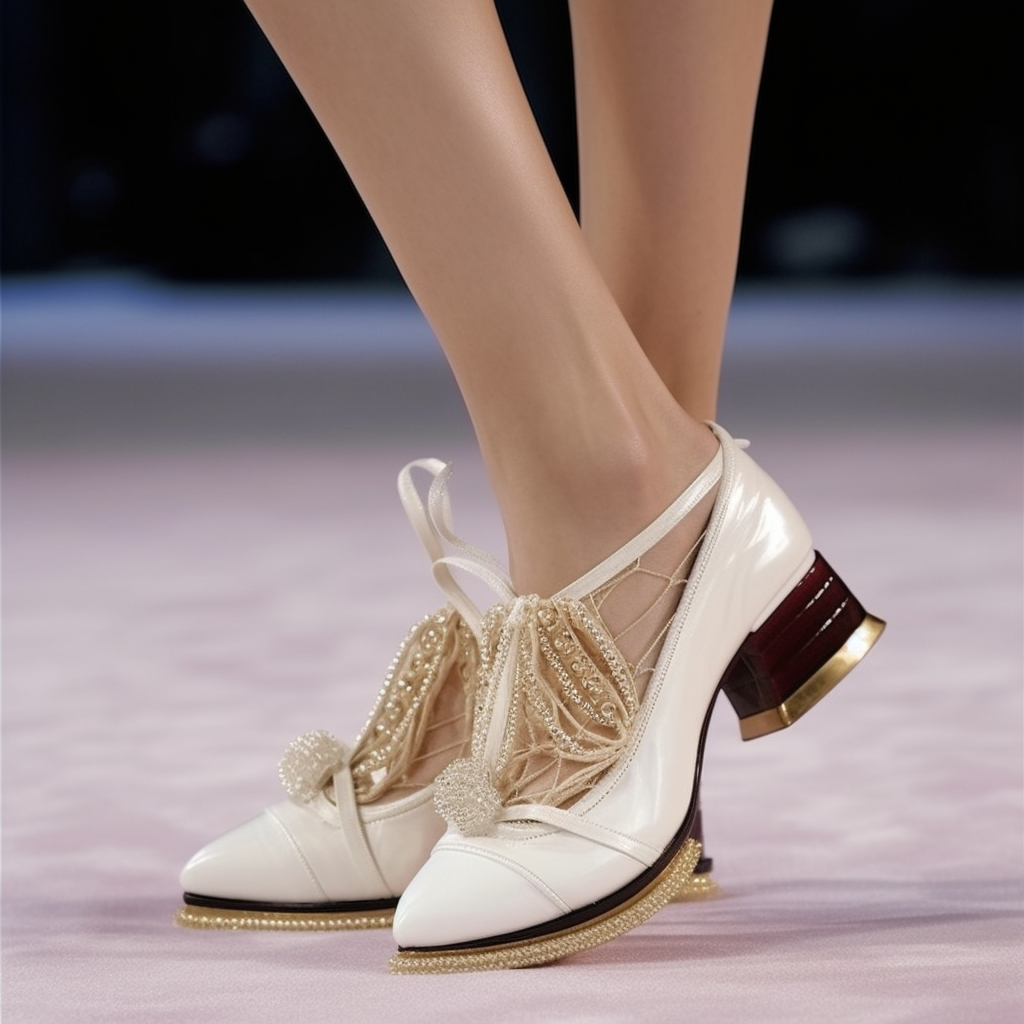The photograph captures the calves of a woman's legs adorned in white, intricately embellished shoes. The focus is primarily on the shoes, which feature low, dark heels with golden banding at the base. The front of the shoes is adorned with a profusion of beading and a pom-pom hanging from the ties. Additionally, the shoes are bound with white ribbons interspersed with gold detailing, and their soles shimmer with a sparkly gold finish. The legs, light tan in color, stand on a light-colored floor against a black, indistinct background, providing a stark contrast that emphasizes the sharpness and intricate details of the footwear.